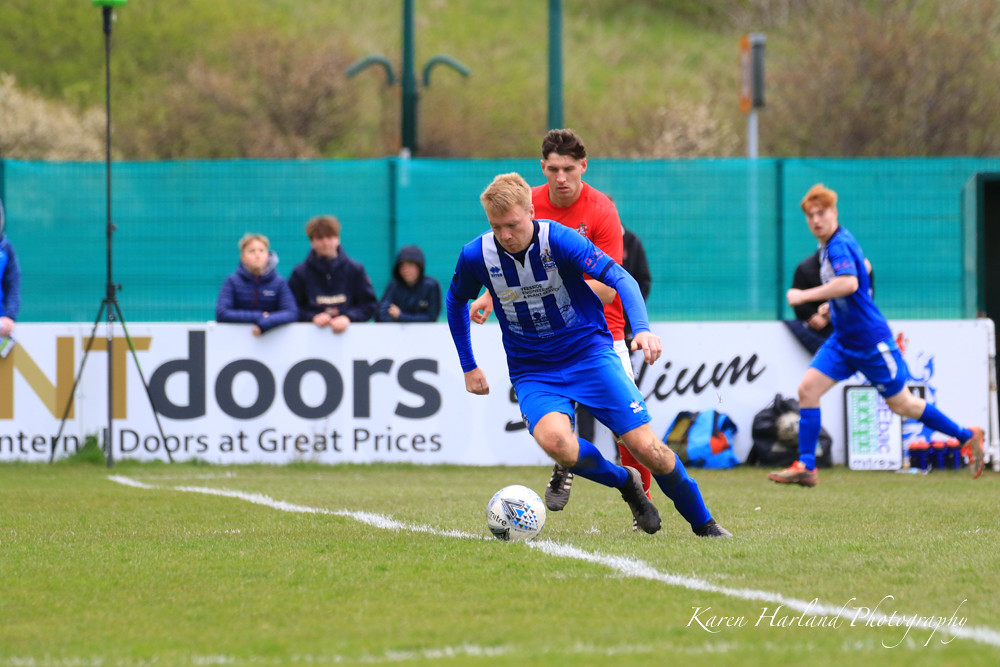This detailed photograph, captured by Karen Harland Photography, depicts a lively scene of a British football match taking place on an outdoor field. At the center of the image, a focused player clad in a blue and white striped jersey, blue shorts, and blue socks, is poised to kick a white football resting on a white line on the field. Just behind him, another player from the opposing team is dressed in a red t-shirt, white shorts, and red socks, while a teammate in the same blue uniform is seen in the right foreground. The sidelines are lined with the players' gear and bags, placed against a white banner that reads "NT Doors, Internal Doors at Great Prices." Spectators, bundled up in coats, lean against this banner as they intently watch the game. Above the spectators, a turquoise barricade separates them from a picturesque backdrop of green trees and shrubs, which includes touches of purple and pale pink. The word "STADIUM" can be discerned in the background, completing this vibrant and dynamic scene.